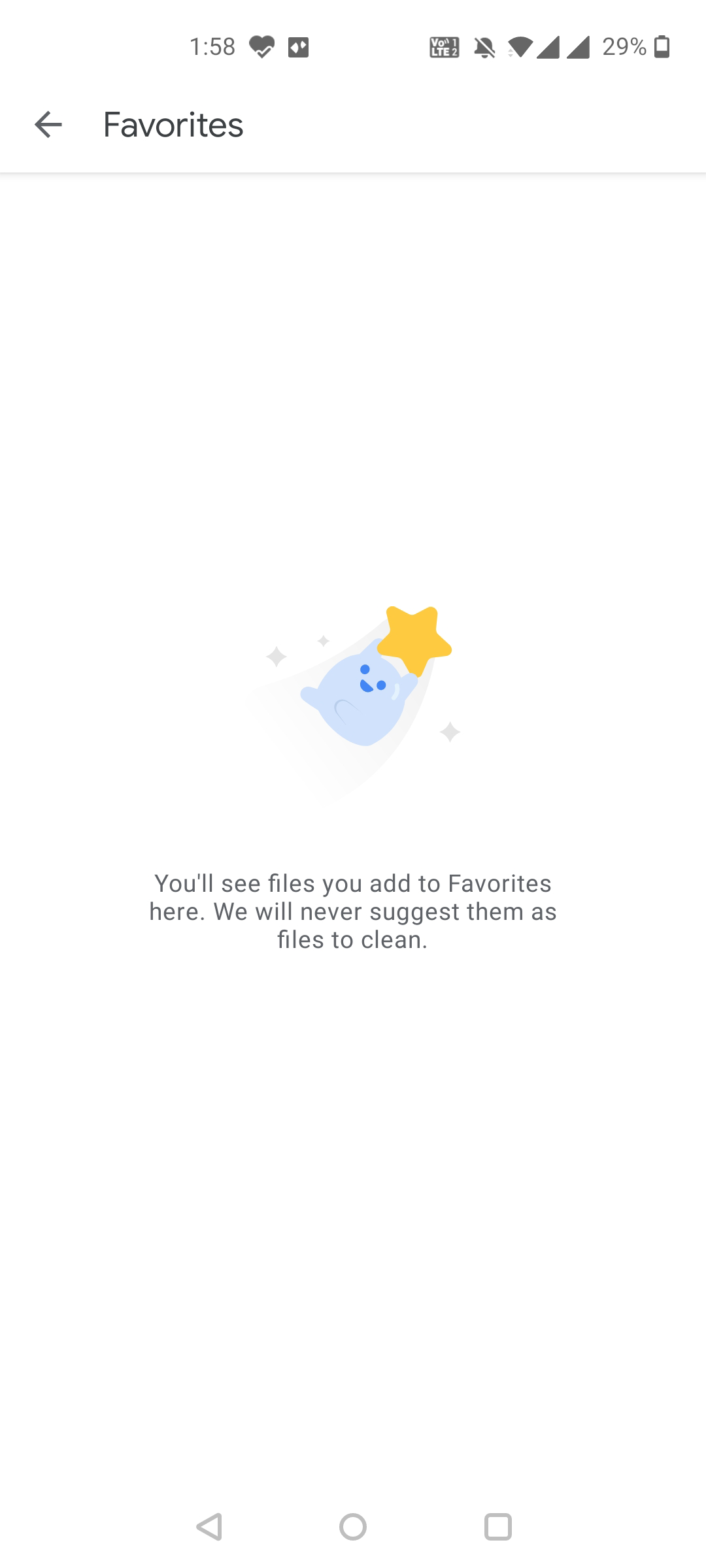Caption: The image is a screenshot taken from a mobile phone displaying a specific app interface. At the top, the status bar shows the time as 1:58 PM, accompanied by a heart symbol and a photo icon. Moving to the right, there is a blank space, followed by more icons including notifications turned off, a rectangular icon, a Wi-Fi symbol, and two triangles. The battery icon shows a 29% charge with an almost empty battery indicator—the majority white with a small black sliver at the bottom.

Below the status bar, there is a navigation arrow pointing to the left next to the word "Favorites," which is underlined by a faint gray line. At the center of the screen, a whimsical creature appears diagonally, holding a star with a golden yellow-orange hue. Beneath this illustration, small gray text reads, "You'll see files you add to favorites here. We will never suggest them as files to clean."

The bottom of the screen features a white background with three navigation icons: a gray triangle pointing to the left, a circle, and a square.